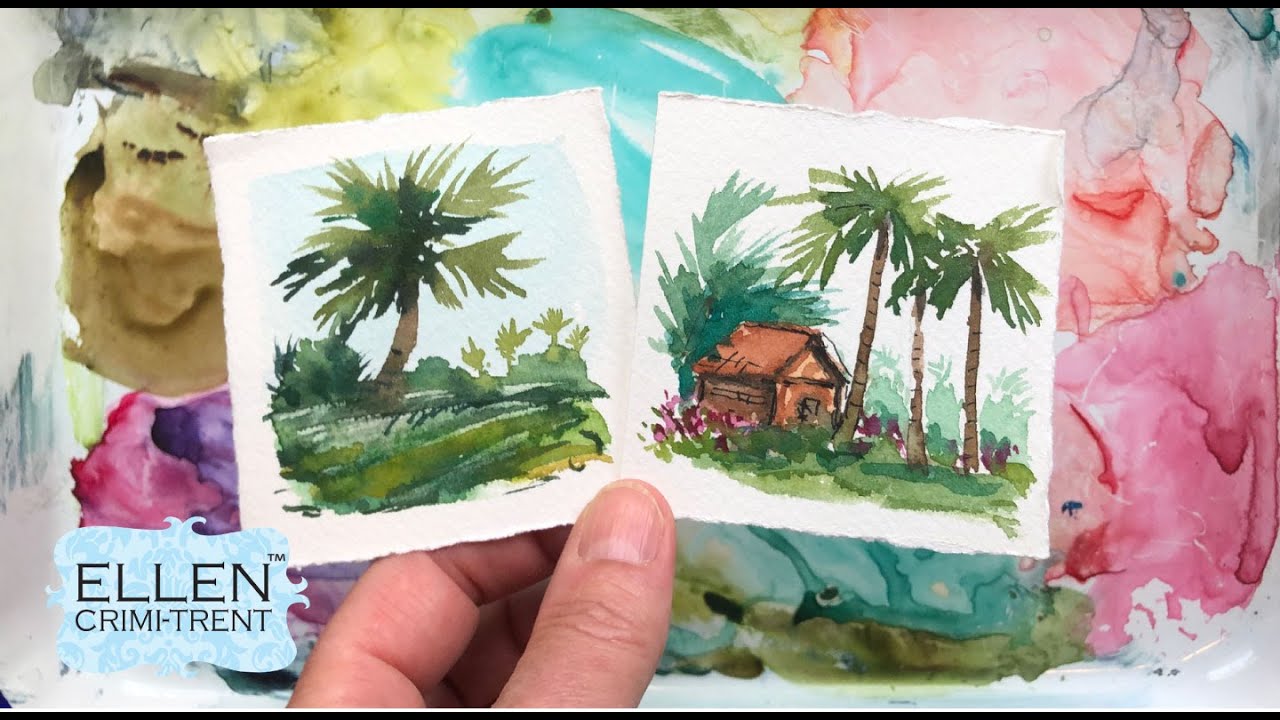The photo depicts a detailed scene where a man's left hand is holding two small, square watercolor paintings with white borders. The painting on the left features a landscape with a green palm tree, lush green grass, distant mountains, and a blue sky. The painting on the right shows a similar scene with multiple palm trees, a small brown cabin, and red flowers in the foreground. Both paintings appear vibrant and meticulously crafted. In the bottom left corner of the image, the signature "ELLEN CRIMI-TRENT" appears in all capital letters, with a small trademark symbol next to it. Beneath these two paintings, the background reveals a larger watercolor composition with colorful swirls and drips in red, yellow, blue, purple, and green hues, suggesting an abstract or expressive style that is partially obscured by the smaller paintings. The image is brightly lit, showcasing the clarity and detail of the artworks.